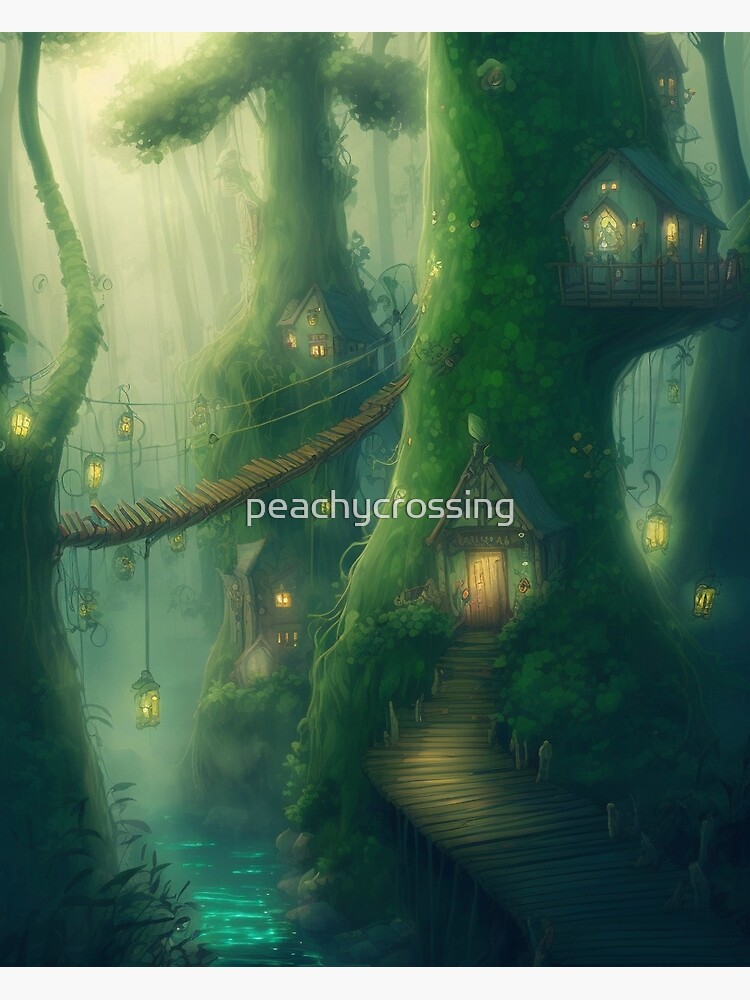In this enchanting, mystical scene titled "Peachy Crossing," we are transported to a secluded, magical forest teeming with life and whimsy. Dominated by towering, moss-covered trees, the forest houses dwellings intricately built into the trunks and branches of these huge, green giants. The central focus is a grand tree with a wooden path that ascends to its entrance, leading to a house that is almost part of the tree itself. Surrounding this tree, more homes are nestled within the branches and connected by a network of wooden bridges adorned with glowing lights, casting a gentle, ethereal glow upon the water below. Lily pads float lazily on the glistening, luminous river that snakes through the scene, adding to the fantastical ambiance. Fireflies drift about, providing natural, twinkling illumination. The landscape is filled with various shades of misty yellows and greens, enhancing the magical, animated quality of the image. At the center, the text "Peachy Crossing" blends seamlessly into this enchanting tableau, marking the artist's whimsical creation.